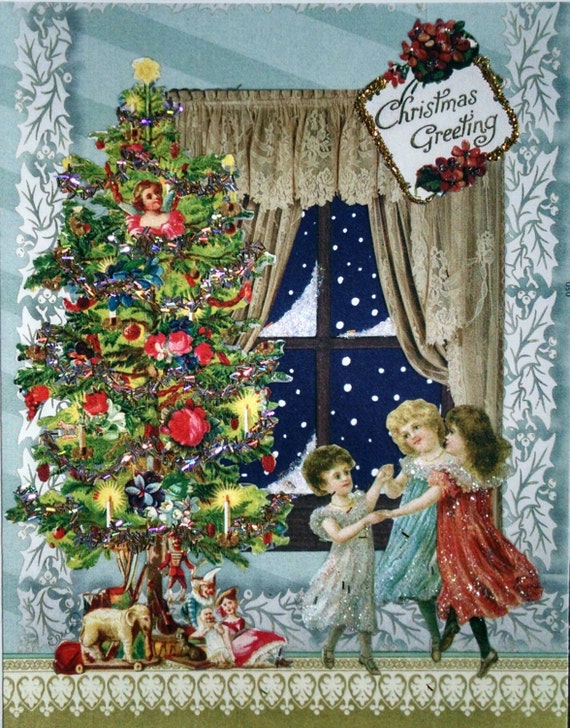This detailed Christmas card features a festive scene centered around a large green Christmas tree, adorned with a star on top and various ornaments, including red circles, flower patterns, and Christmas lights reminiscent of candles. The tree is situated to the left side of the card, and beneath it, there are various toys, including an elephant riding a skateboard, an action figure, a dog, small dolls, and perhaps a car. A colorful border made up of light blue leaves frames the entire card. 

In the background, there's a sizeable window with slightly opened dark brown curtains through which a dark blue night sky filled with falling snowflakes is visible. In the top right corner of the window, a small square label displays the words "Christmas Greeting" in black lettering, adorned with bows on both the top and bottom.

In the forefront, three little girls hold hands and dance in a circle. The girl on the left, with short brown hair, is dressed in a glittering white dress with gray slippers. The girl to the right, slightly behind her, has blonde hair and wears a shimmering blue dress. The third girl, positioned with her back to the right, faces the left girl, sporting a red dress, black tights, and black shoes. The joyful scene captures the essence of Christmas, with its serene snowy backdrop and lively festive elements.